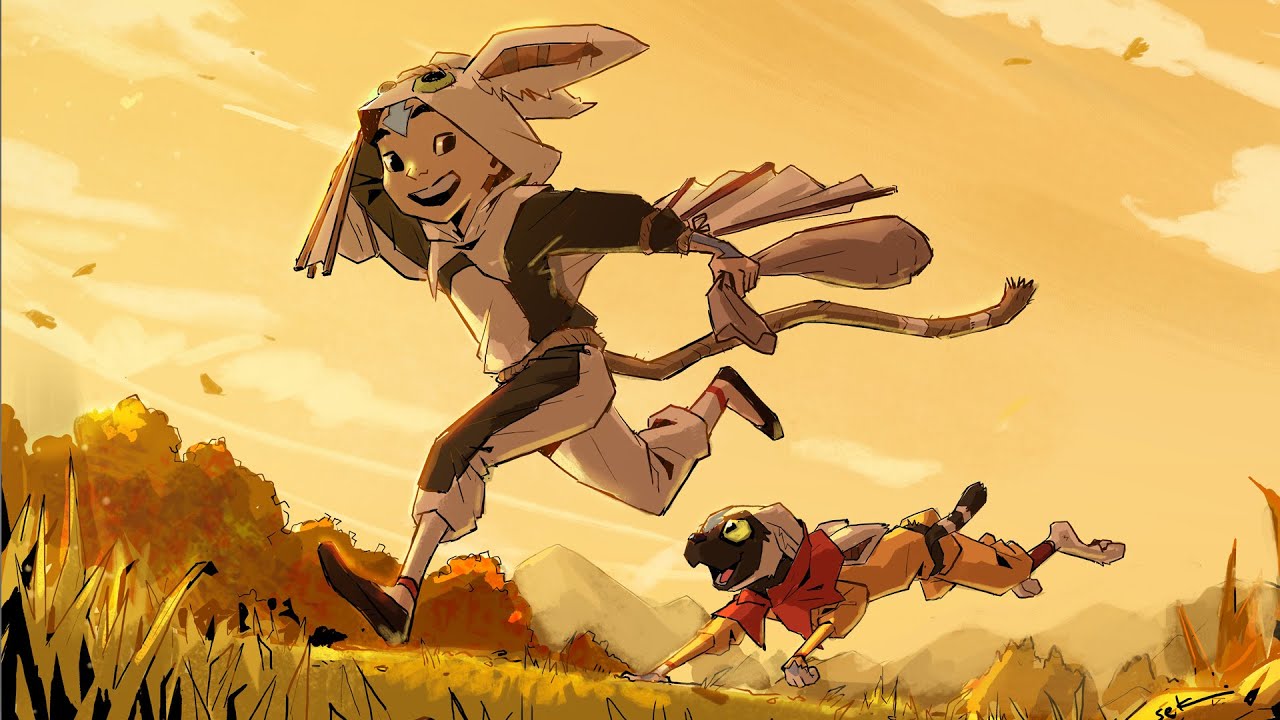The image is a stylized cartoon or anime drawing depicting a scene set during an autumn dusk with two characters running through a field. The sky is a gradient of faded orange and yellow with scattered clouds mostly on the left and right sides. In the background, there are gray mountains and a mix of orange, yellow, and red bushes that add to the fall ambiance. The grass is light green interspersed with patches of orange.

The main character appears to be a child of indeterminate gender wearing a rabbit-themed headpiece with visible ears and eyes. They have brown hair peeking out from under the hoodie. They are dressed in white clothing with black splotches around the arms and the tops of the legs, which are capri-length, and they wear brown sandals or shoes. A cyan-colored arrow points downward on their forehead, ending just below their eyebrows. The child has a smile on their face and seems to be holding a sack.

Running beside the child is a dog that is brown with white feet and yellow ears. The dog is donning a red shirt and orange-yellow pants, which are part of a jumpsuit-like outfit. The canine's tail is striped brown and cream. Both characters are moving across the field as they are enveloped in the warm, autumnal color scheme of the setting.